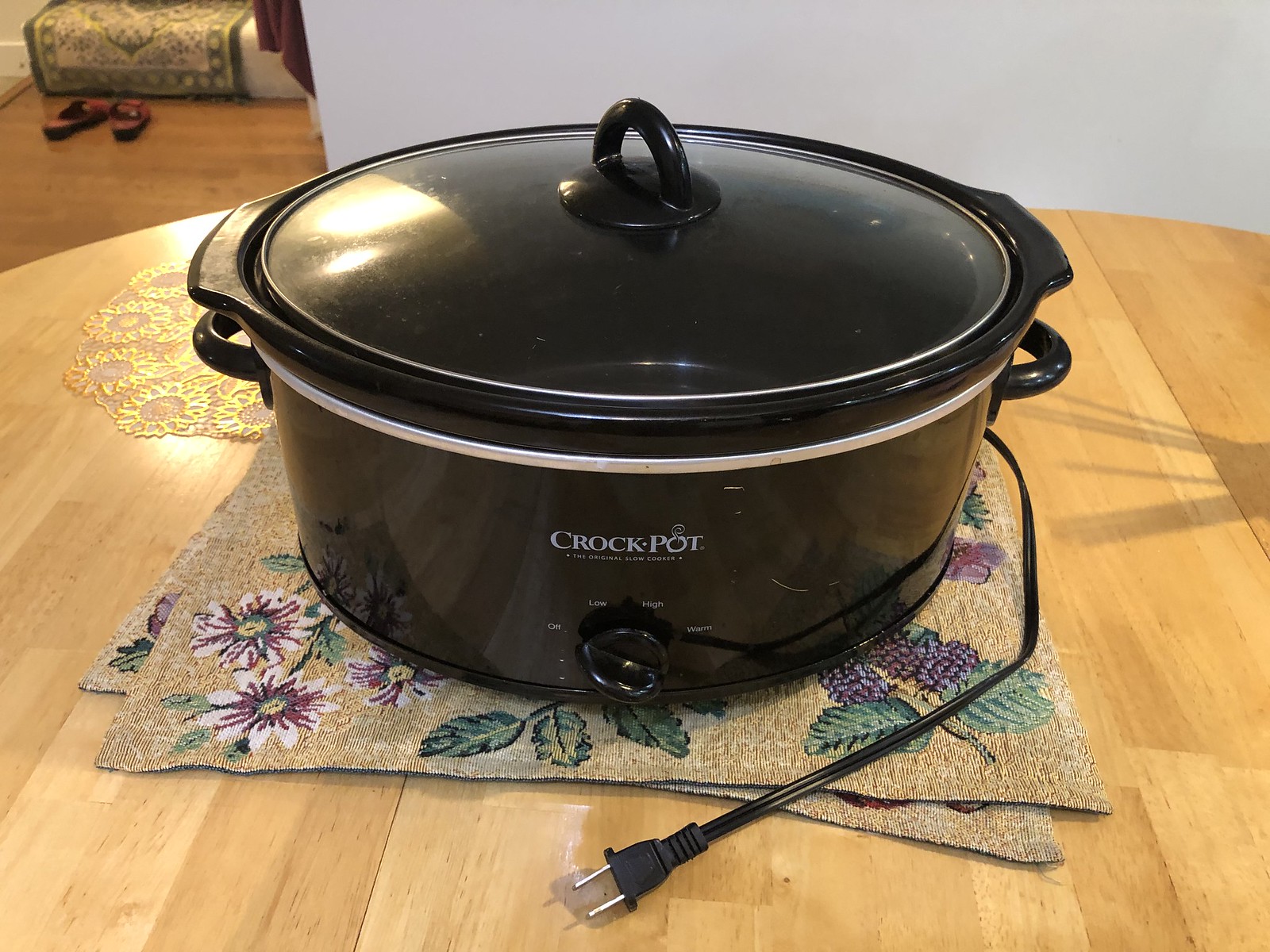This detailed photograph captures a black crockpot resting on a light brown-yellow, wooden circular table. The table is adorned with beige placemats featuring a floral and fruit pattern, including purple grapes, green leaves, and pink flowers. The crockpot, labeled "Crockpot" in white text on its front, has a black dial with small white labels for settings: "off," "low," "high," and "warm." A black electrical cord extends from the side of the crockpot, wrapping around towards the front. The crockpot is equipped with a basin for cooking and heating food, covered by a glass lid with a black plastic handle. In the background, there is a white wall, more wooden floor, a pair of brown slippers on the far left, and a green rug with a possible floral pattern.